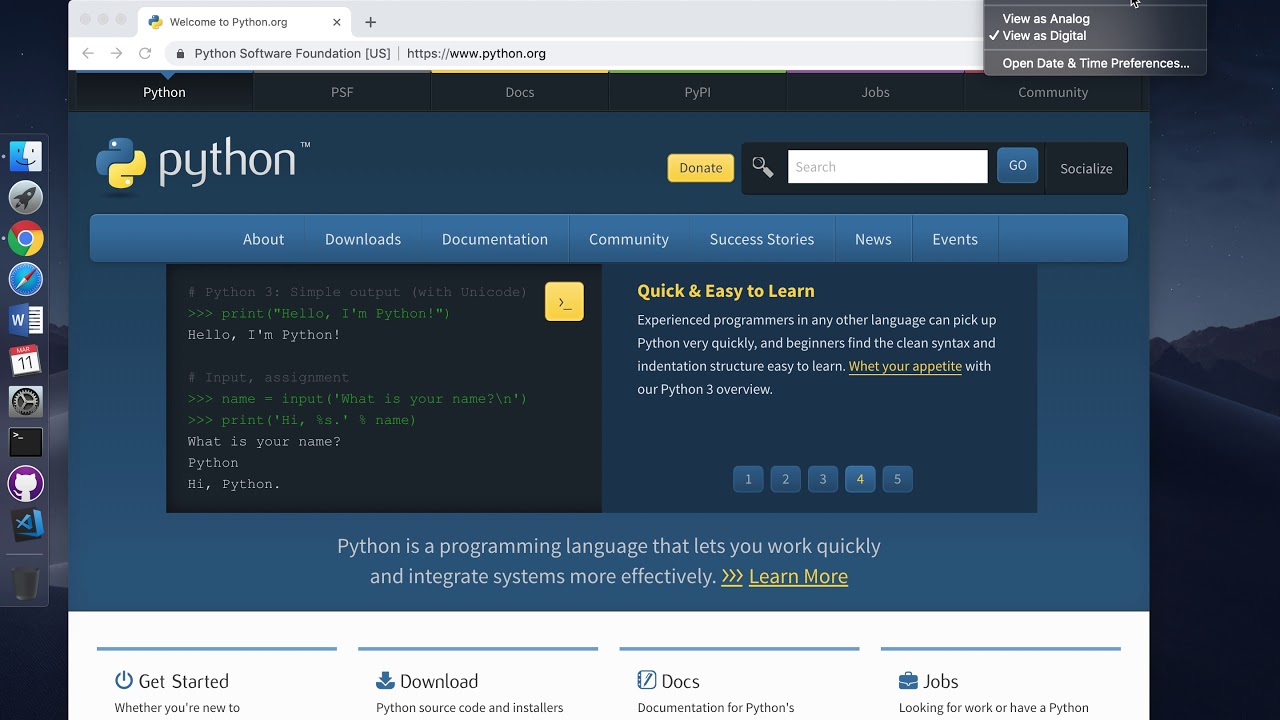The image showcases the homepage of the Python Software Foundation's website, accessible via the URL www.pythonsoftwarefoundation.python.org. The website design features a dark background with a navigation bar at the top, segmented into several tabs: Python, PSF, Docs, PYPI, Jobs, and Community. The "Python" tab is highlighted in white, indicating the active section, while stores are mentioned on the top right in grey.

Dominating the main page is the Python logo, which consists of two stylized python snakes forming a shape reminiscent of the initials 'Py'. The top snake is colored blue and the bottom one orange, both sporting white eyes. The word "Python" accompanies the logo in white text.

To the right of the logo, there is a gold-colored search button. Adjacent to it on the left, there is an orange "donate" button. Further down, a secondary navigation bar also set against a dark blue background includes the following links in white text: About, Download, Documentation, Community, Success Stories, News, and Events. 

Prominent on the right side is a highlighted yellow text box stating, "Quick and easy to learn." Below this, additional text explains, "Experienced programmers in any other language can pick up very quickly, and beginners find the clean syntax and indentation structure easy to learn. Whet your appetite with our Python 3 overview."

Below this introduction, there are pagination indicators numbered 1 through 5, with 4 being currently selected. On the left, an example Python code snippet is displayed, saying:
```python
print("hello I'm Python")
hello I'm Python
what is your name?
Python
hi Python
```

Towards the bottom of the page, there is an explanatory text stating, "Python is a programming language that lets you work quickly and integrate systems more effectively." There is also an "Learn more" link highlighted in orange.

At the very bottom, there are various quick access links such as "Get started," "Python source code and installers," "Documentation for Python," and a notice about "Looking for work or have a Python."